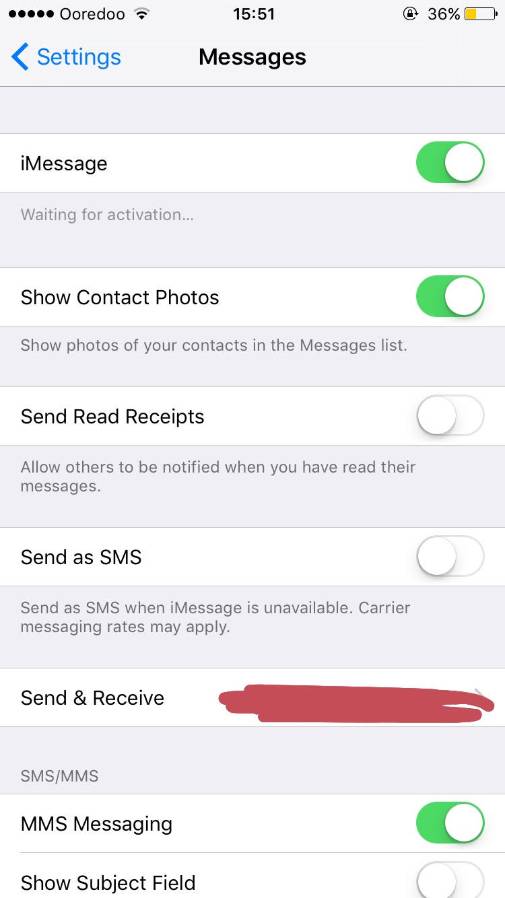A screenshot of the iMessage settings page on an iPhone. The settings menu lists various options with the following statuses:
- "Show Contact Photos" toggle is enabled.
- "Send Read Receipts" toggle is disabled.
- "Send as SMS" toggle is disabled.
- Option to choose where to send and receive messages has strikethrough text.
- "MMS Messaging" toggle is enabled.
- "Show Subject Field" toggle is repeatedly shown as disabled.